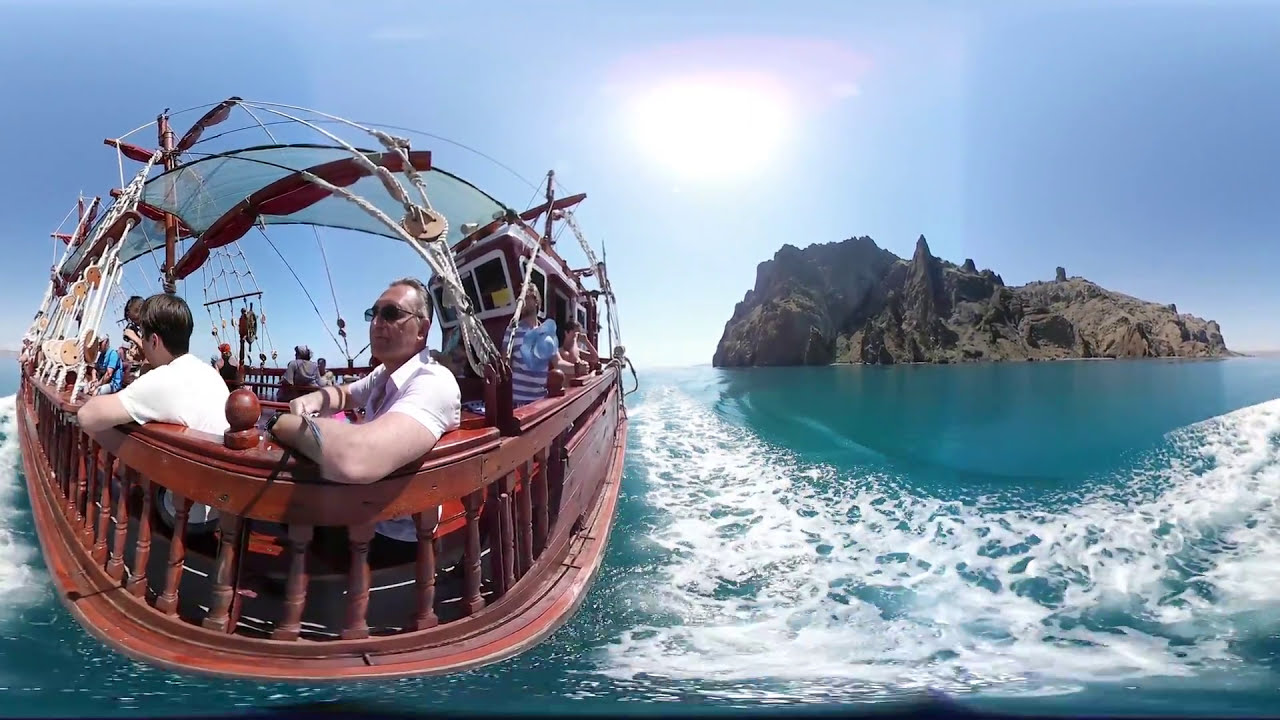The photograph captures a vibrant outdoor scene on a bright, sunny day. Dominating the center of the image is a rugged, rocky island, devoid of plant life, with its jagged edges sharply outlined against the clear blue sky. The sun shines brilliantly above the island, casting a glowing white light across the scene. Below the island, the water stretches out in a serene expanse of blue, though it appears greenish in some areas, until it becomes frothy and wavy toward the foreground, stirred by the wake of a boat.

On the left side of the photo, a wooden sailboat, with dark wood-colored railings, appears slightly distorted due to the angle of the photograph. The boat is populated by several passengers, numbering between seven and eight, most of whom are seated. Notably visible is an older man in a white short-sleeved shirt and sunglasses, possibly resting his arms on the railing. Next to him, another man, likely younger, also dons a white shirt. The boat's movement creates a trail of foamy water, adding dynamism to the scene. Overall, the main colors of the photograph are vivid hues of blue, green, brown, tan, and white, creating a strikingly clear and detailed portrayal of this tranquil maritime moment.